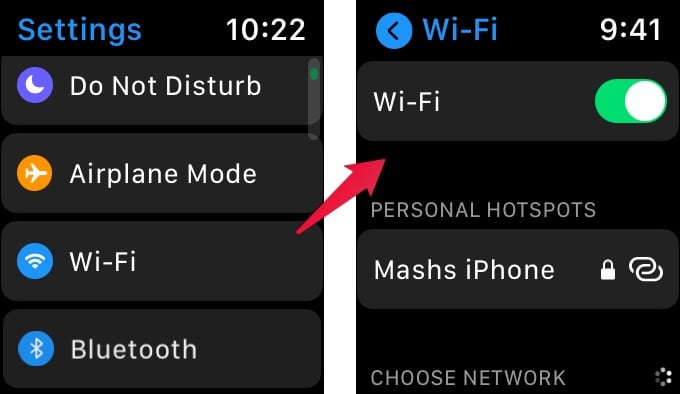This split image visually guides the user through a two-step process for activating a personal hotspot on an iPhone. The left image displays the initial screen, showcasing the settings menu on a dark background, with the time '10:22' displayed in the upper right-hand corner. In the upper left, the word "Settings" is prominently featured. Below it, four categories are listed with corresponding icons: "Do Not Disturb" (moon icon), "Airplane Mode" (airplane icon), "Wi-Fi" (traditional Wi-Fi icon), and "Bluetooth" (traditional Bluetooth icon). A red arrow, Photoshopped in for emphasis, directs the viewer's attention from the "Wi-Fi" option to the second image on the right.

The second image under the same black background indicates the Wi-Fi settings screen at a different time, '9:41'. Here, the Wi-Fi is shown as toggled on, indicated by the green switch. Beneath this, a section titled "Personal Hotspots" lists "Mashes iPhone" which is secured with a lock icon, and has an option to connect. This step-by-step visual guide makes the process of setting up a personal hotspot both intuitive and straightforward.